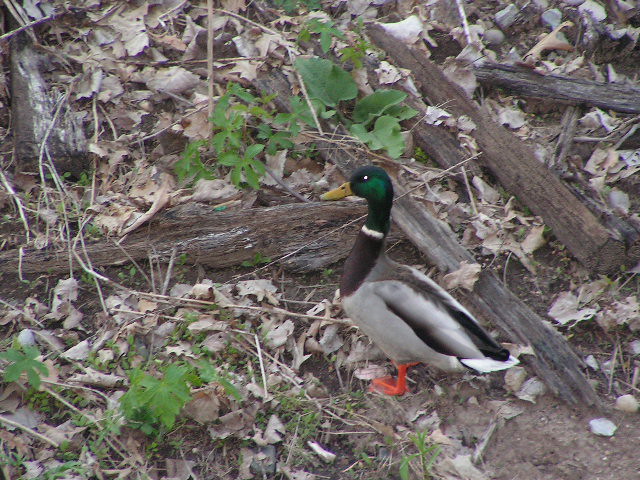A bright orange-footed mallard duck, featuring its characteristic iridescent green head, yellow beak, and a distinctive white neck ring, is captured in a side view as it gazes to the left. Its chest and wings display a spectrum of colors ranging from brown and grey to white and black. The duck is seen walking in a forest-like setting, amidst a scattering of broken branches, wood chunks, and twigs. The ground is littered with dead, brown leaves, interspersed with patches of green grass, weeds, and small shrubs. Additionally, there are some stones and dirt forming a natural backdrop for this serene wildlife scene.